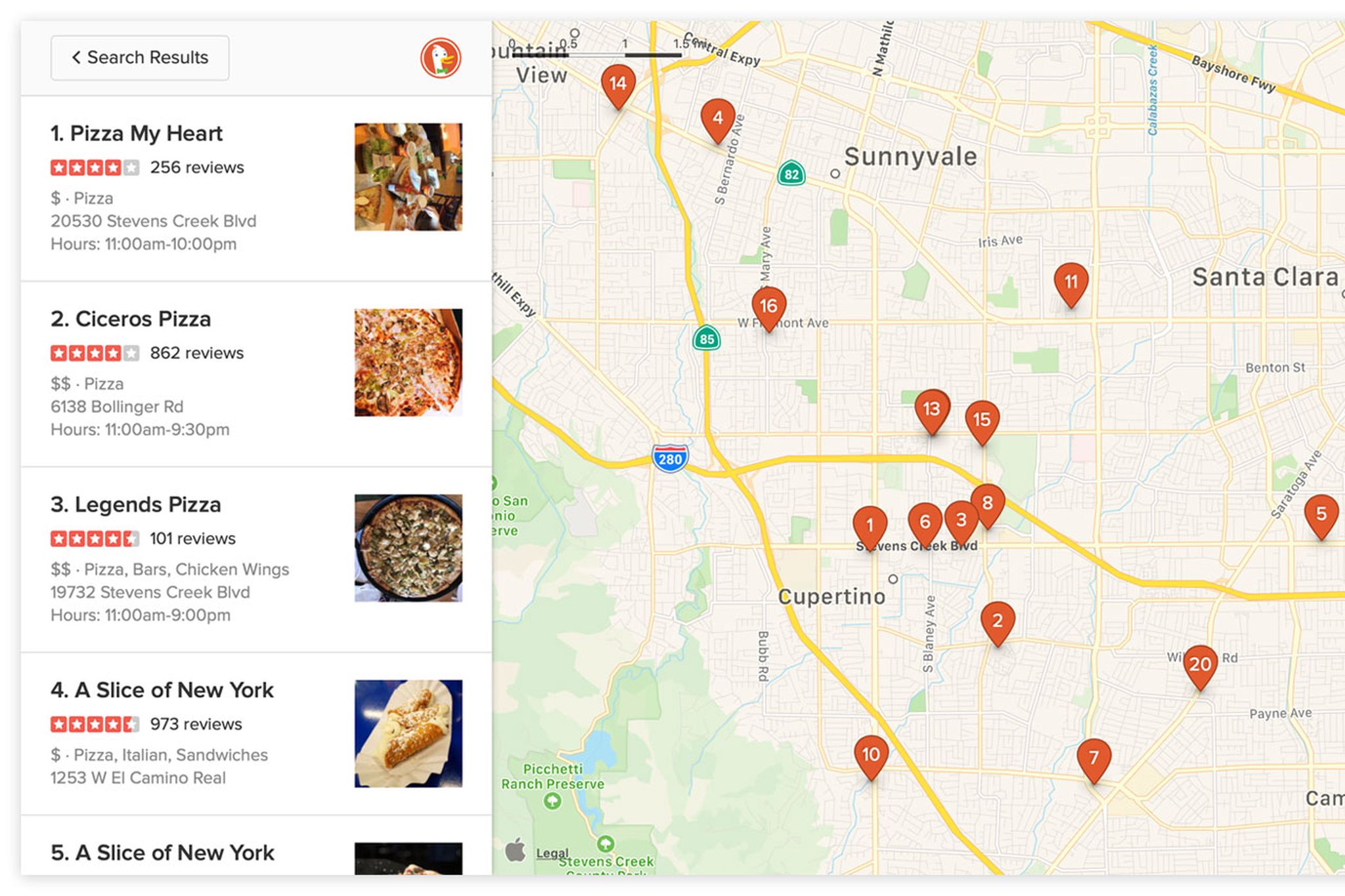This image depicts a detailed map of California's Bay Area, specifically highlighting the cities of Sunnyvale, Santa Clara, and Cupertino. The map features a series of 16 numbered red pins, each representing a distinct food establishment, likely pizzerias. 

On the left side of the map, there is a numbered list correlating with the pins, providing names and images of the featured pizzerias:
1. **Pizza My Heart** – The image shows a pizza with hues of orange, brown, and red, though the details are somewhat unclear.
2. **Cicero's Pizza** – Accompanied by a clearer image of a pizza.
3. **Legends Pizza** – Features a darker pizza, suggesting it is heavily topped, possibly with meats.
4. **A Slice of New York** – Displays a folded slice of pizza, indicative of New York-style pizza.
5. **A Slice of New York (again)** – This entry is partially cut off, making the pizza slice difficult to see. 

The detailed map visually organizes and highlights these local pizzerias for easy reference.